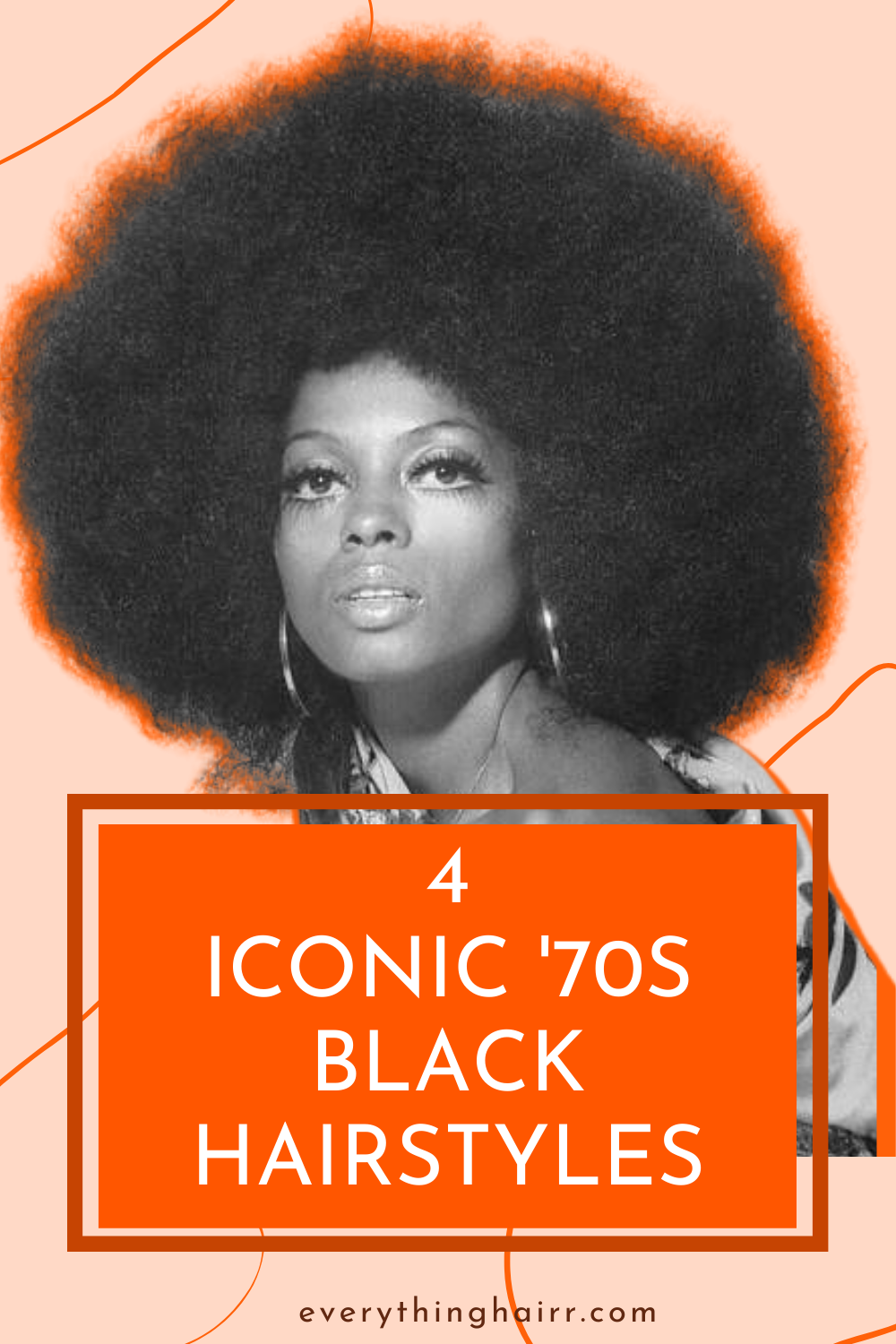This image features an African-American woman who closely resembles the singer Diana Ross. She is looking forward and flaunts a significantly large, poofy Afro hairstyle, with her black hair framed by a slight orangish aura that enhances its boldness. She is adorned with big hoop earrings and a hint of lipstick, adding to her elegant appearance. The background is a light orange, almost peach or salmon in color, accentuated with randomly placed orange streaks that add visual flair. At the bottom of the image, within an orange rectangle bordered by a darker red shade, white text reads, "Four iconic 70s black hairstyles," and just below this, in black text, it says, "everythinghair.com," with a playful double 'R' in "hair." The photo overall gives the impression of being a magazine cover or an advertisement, celebrating iconic 1970s black hairstyles.